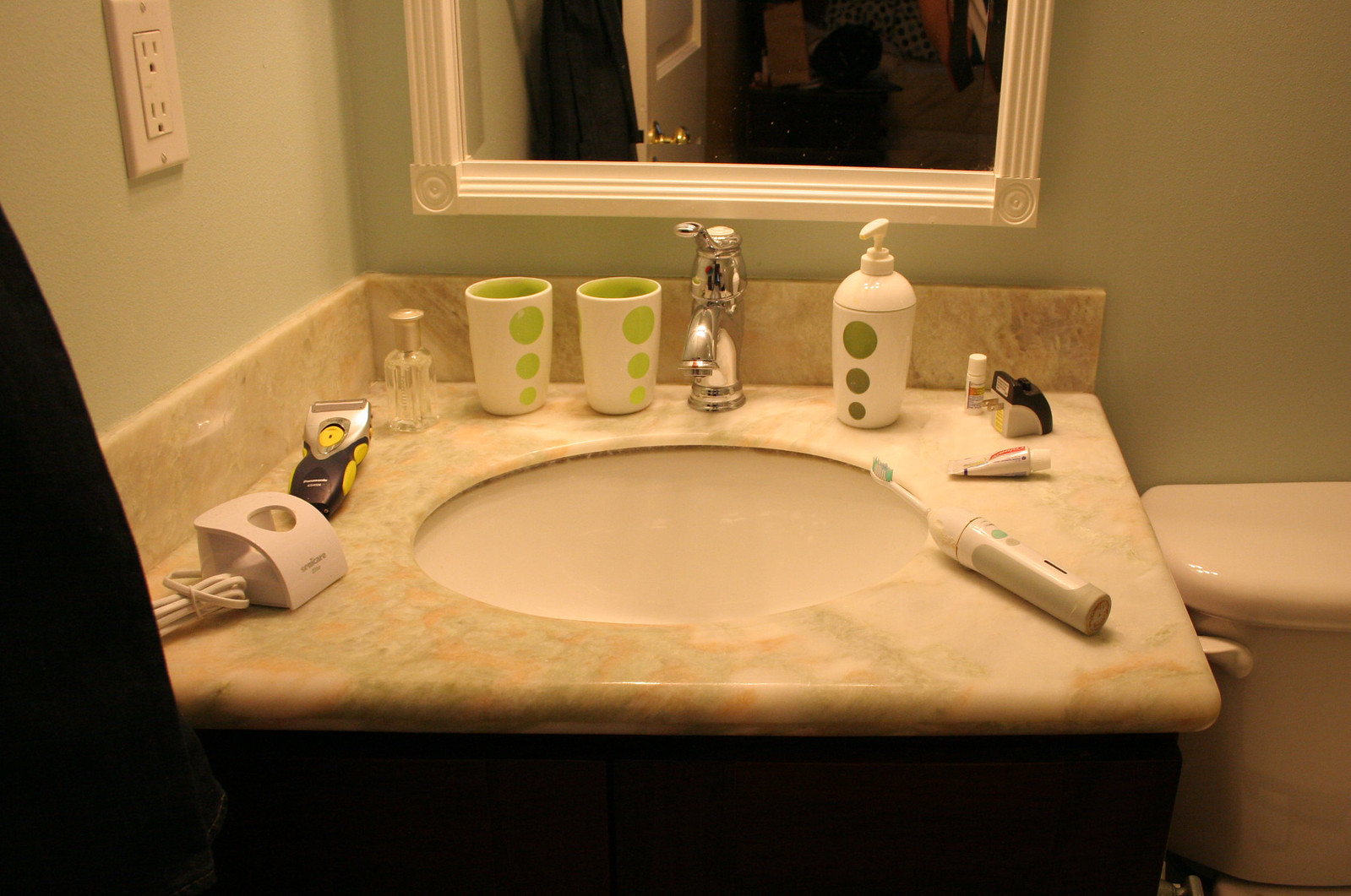This image showcases a compact, 24-inch square bathroom vanity countertop with a simple, standard sink. The countertop sink is accompanied by a sleek, silver spout featuring an integrated lever handle for adjusting water temperature, rather than separate knobs. To the left of the faucet, two pristine white cups decorated with three graduated light green circles - a large one on top, a medium in the middle, and a small circle at the bottom - neatly sit. The inside of these cups is the same vibrant green as the circles on the exterior. In the corner of the vanity, a small clear glass perfume bottle with a silver cap stands on a matching backsplash, elegantly complementing the countertop.

Along the left wall, a set of professional-looking silver and black hair clippers with yellow buttons rest beside a plug-in wall charger, which holds the clippers upright. On the opposite side of the sink, an electric toothbrush precariously balances over the open sink edge. Nearby, a small travel-sized toothpaste tube and several indistinct small items, such as a bottle or tube, are scattered. 

To the far right, just the top portion of a beige porcelain toilet tank is visible, with its handle on the extreme left side. Above the vanity, an 8-inch section of a white-framed wall mirror reflects an open white door. Adjacent to the mirror on the left wall, there's an unoccupied GFI bathroom outlet above the countertop, set against a backdrop of pale green painted walls.